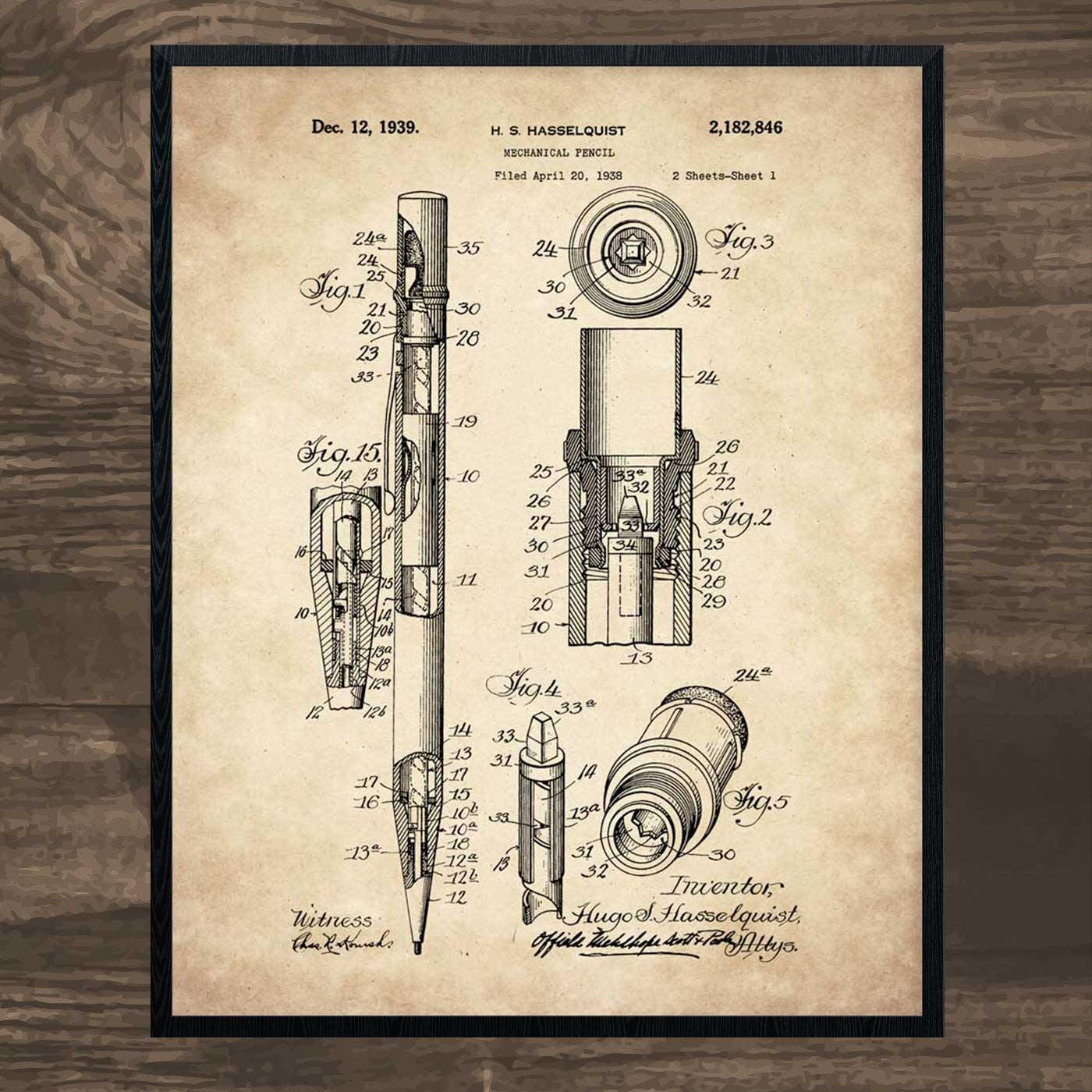This detailed image showcases a meticulously drawn and labeled patent diagram for a mechanical pencil invented by H.S. Hasselquist. The document, dated December 12, 1939, with a filing date of April 20, 1938, bears the patent number 2,182,846. At the top center, "H.S. Hasselquist Mechanical Pencil" is typed in tiny black letters. The diagram prominently features the pencil in a vertical orientation, exposing its internal components, each meticulously numbered. To the right, various sectional views illustrate the top, middle, chamber, and tip of the pencil. The bottom left corner of the document includes a witness signature, while the bottom right bears the signature of Hugo S. Hasselquist, the inventor. This piece of historical engineering is framed in a thin black frame and rests on an ashy-colored wooden table, highlighting the aged white paper and the intricacy of the black ink etching that captures every component of the mechanical pencil in fine detail.